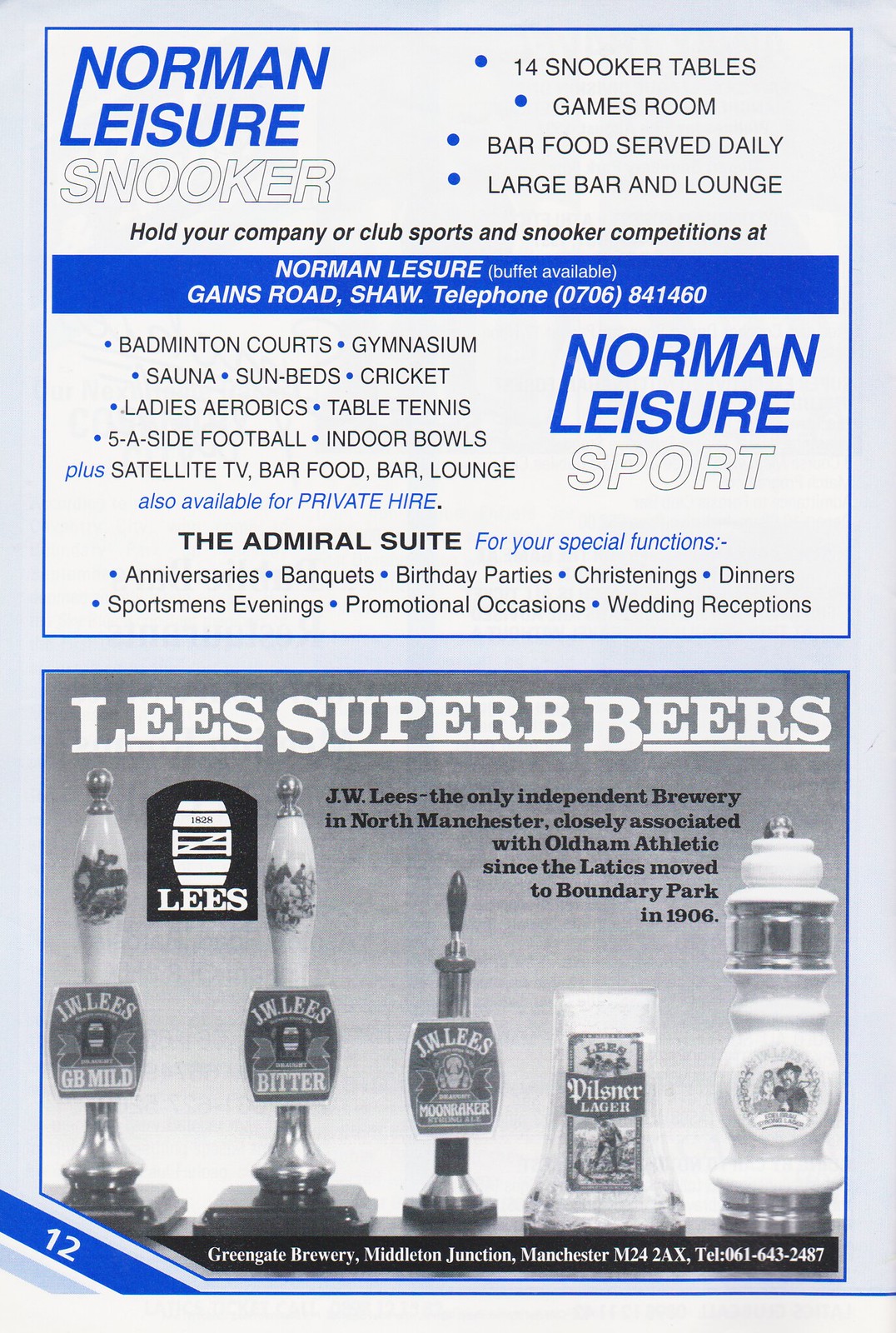This image features a scan from a vintage sports program or magazine, showcasing two distinct advertisements on a single page, specifically page 12, as indicated by the blue number in the bottom left corner. The top half of the page prominently displays an advertisement for Norman Leisure Snooker. The ad, set against a white background with blue accents, encourages businesses and clubs to host their sports and snooker competitions at Norman Leisure. It highlights additional amenities such as sunbeds, indoor bowls, games rooms, and daily bar food service, also mentioning availability for special functions like anniversaries and wedding receptions.

The bottom half of the page features an ad for Lee's Superb Beers, showcasing the offerings from J.W. Lee's brewery. The black-and-white images depict bar taps and varieties of drinks including J.W. Lee's Bitter, J.W. Lee's GB Mild, and Pilsner lager. The ad emphasizes that J.W. Lee's is the only independent brewery in North Manchester and mentions its long-standing association with old-time athletics, notably since the Latics moved to Boundary Park in 1906. Additionally, it promotes the brewery's location at Greengate Brewery in Middleton Junction, Manchester, and provides contact information. Both advertisements suggest a strong local connection to the Manchester area in England.